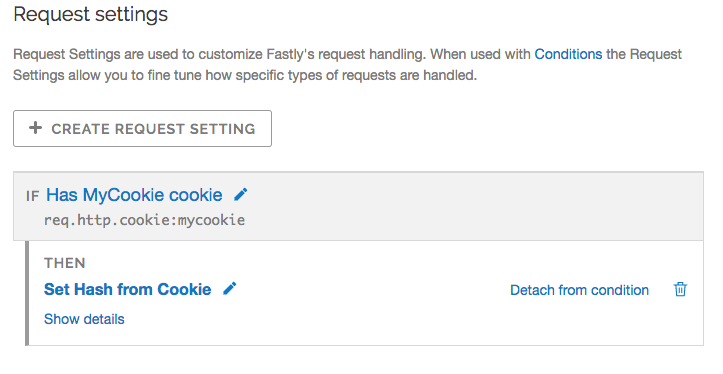A cropped screenshot of a web page illustrating the "Request Settings" section is displayed. The image showcases a white background with predominantly gray text, punctuated by select elements in blue. The content of the screenshot is neatly aligned to the left side of the image, starting from the top and extending downward.

In the main section, the heading "Request Settings" is prominently featured. Below, a description explains that these settings are used to customize Fastly's request handling; when combined with conditions, they allow for fine-tuning the management of specific types of requests. Beneath the explanatory text, a box with the label "Create Request Settings" accompanied by a plus mark is present.

Further down, there is an if-then function described as: "If has my cookie cookie, then set hash from cookie." Options to show details and edit the function using a pencil icon are available. Additionally, a trash bin icon allows for detaching the condition from the function. The overall aesthetic is minimalistic with no additional objects or decorative elements, focusing purely on the functional text within a white space.